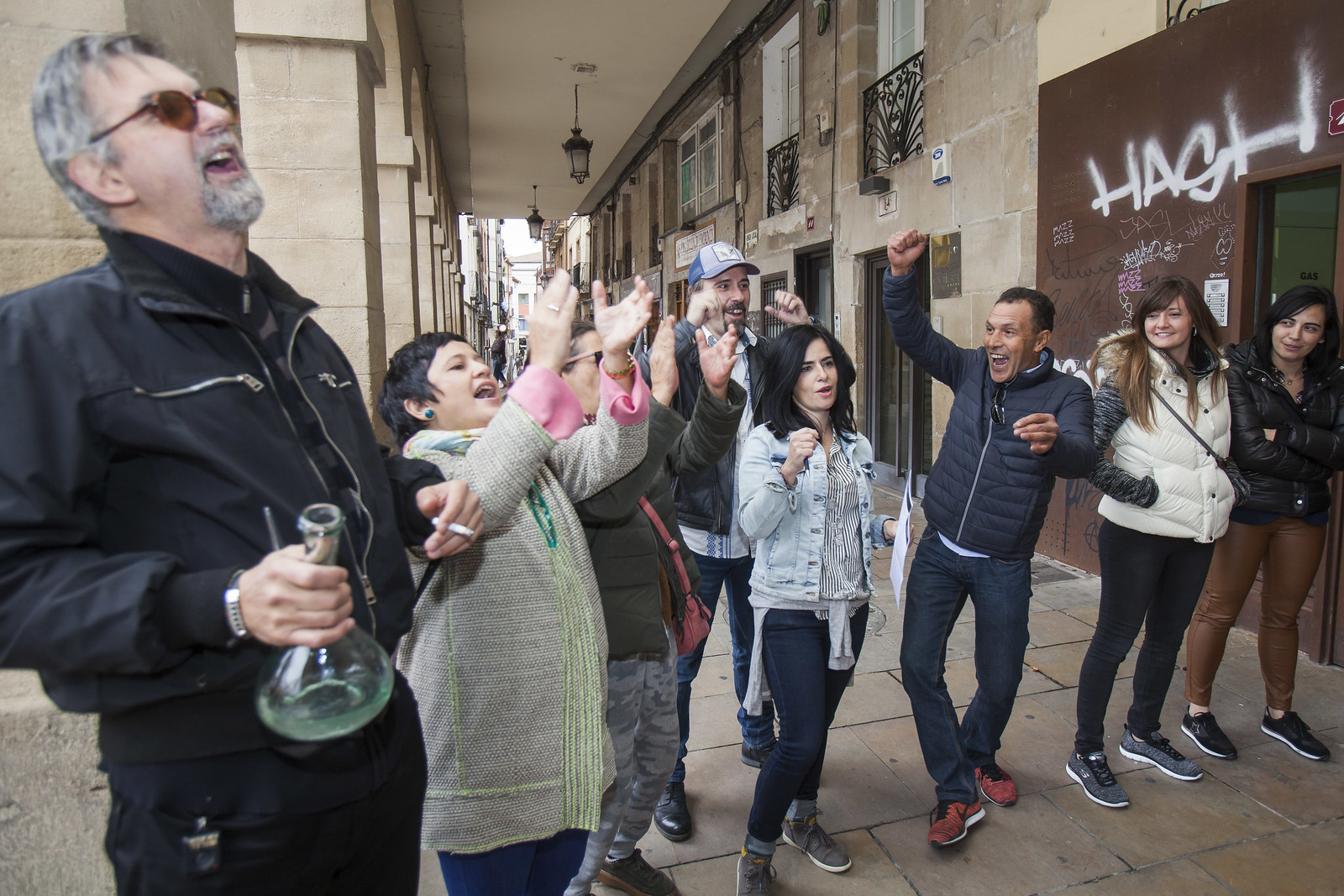The photograph captures a lively outdoor celebration on a city street, in front of a row of storefronts within an old building featuring an open-air breezeway and a concrete awning. Approximately two dozen diverse individuals, dressed in winter outerwear including coats, vests, and sweaters, are gathered in the scene. They all are cheering, clapping, and raising their hands in various expressions of joy and excitement. Central to the group is a young woman in a denim shirt, looking impressed, and beside her is a man in a coat, jubilantly raising his fists and shouting. Another enthusiastic man stands behind him, while a woman in a sweater smiles and claps nearby. To the left, a man in a black jacket and sunglasses joins the revelry, holding a beaker-like glass and a cigarette. The collective attention of the crowd seems focused upwards, suggesting the unveiling or grand opening of a business, given the celebratory atmosphere and the setting among bustling storefronts. The energy of the scene is infectious, with every individual beaming and engaged in the shared moment of joy.